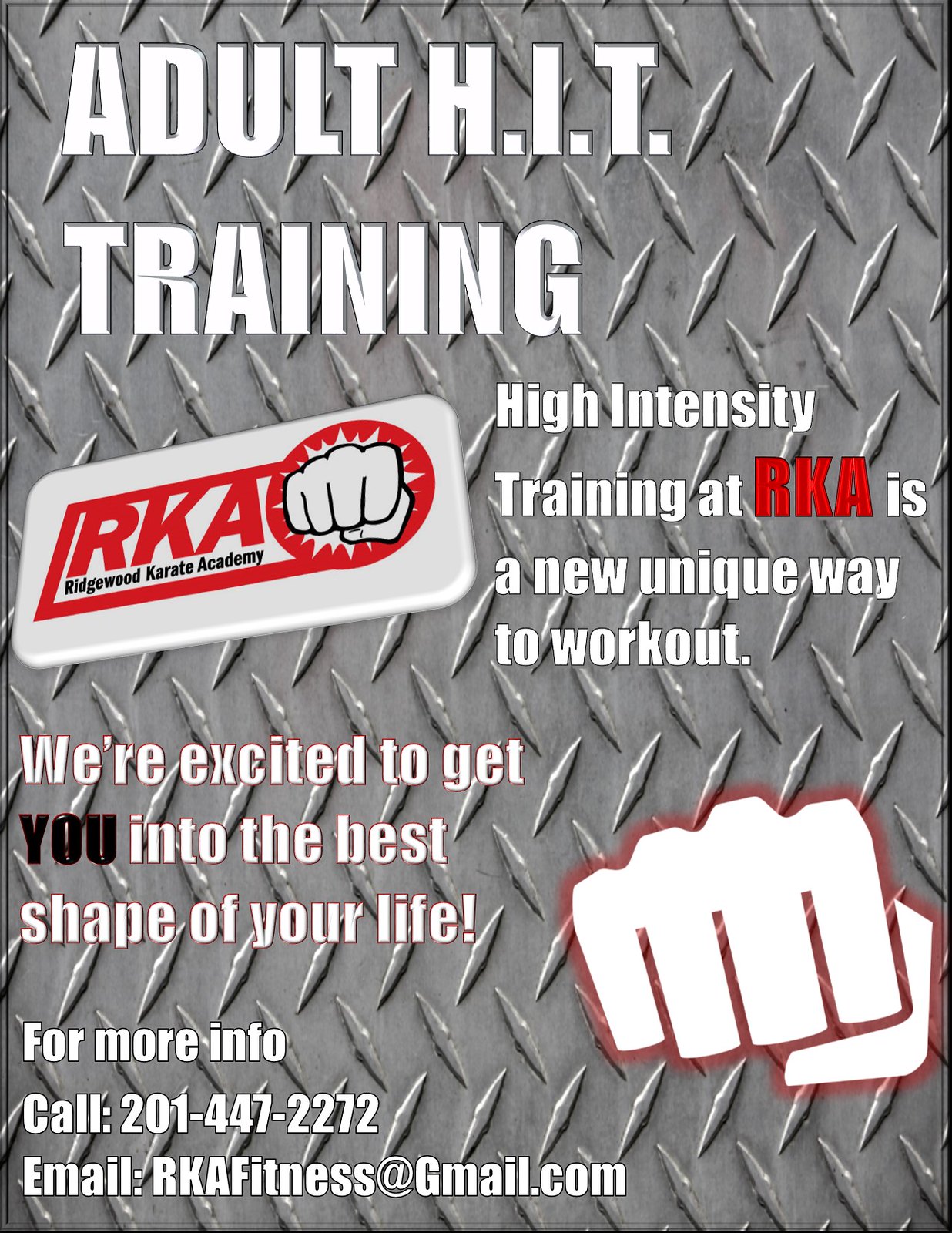The image features a promotional graphic on a textured steel plate background with diagonal lines, reminiscent of the interior of a tractor trailer. At the top, large white text reads "Adult HIT Training." Below that, it states, "High Intensity Training at RKA is a new unique way to work out." To the left, within a rounded rectangle, are the initials "RKA" in red, alongside the full name "Ridgewood Karate Academy" in black. Adjacent to this name is a red logo featuring a black and white fist. At the bottom right of the graphic, another white fist is depicted with glowing red edges. Additional text in white informs, "We're excited to get you into the best shape of your life. For more info, call 201-447-2272 or email rkafitness@gmail.com."